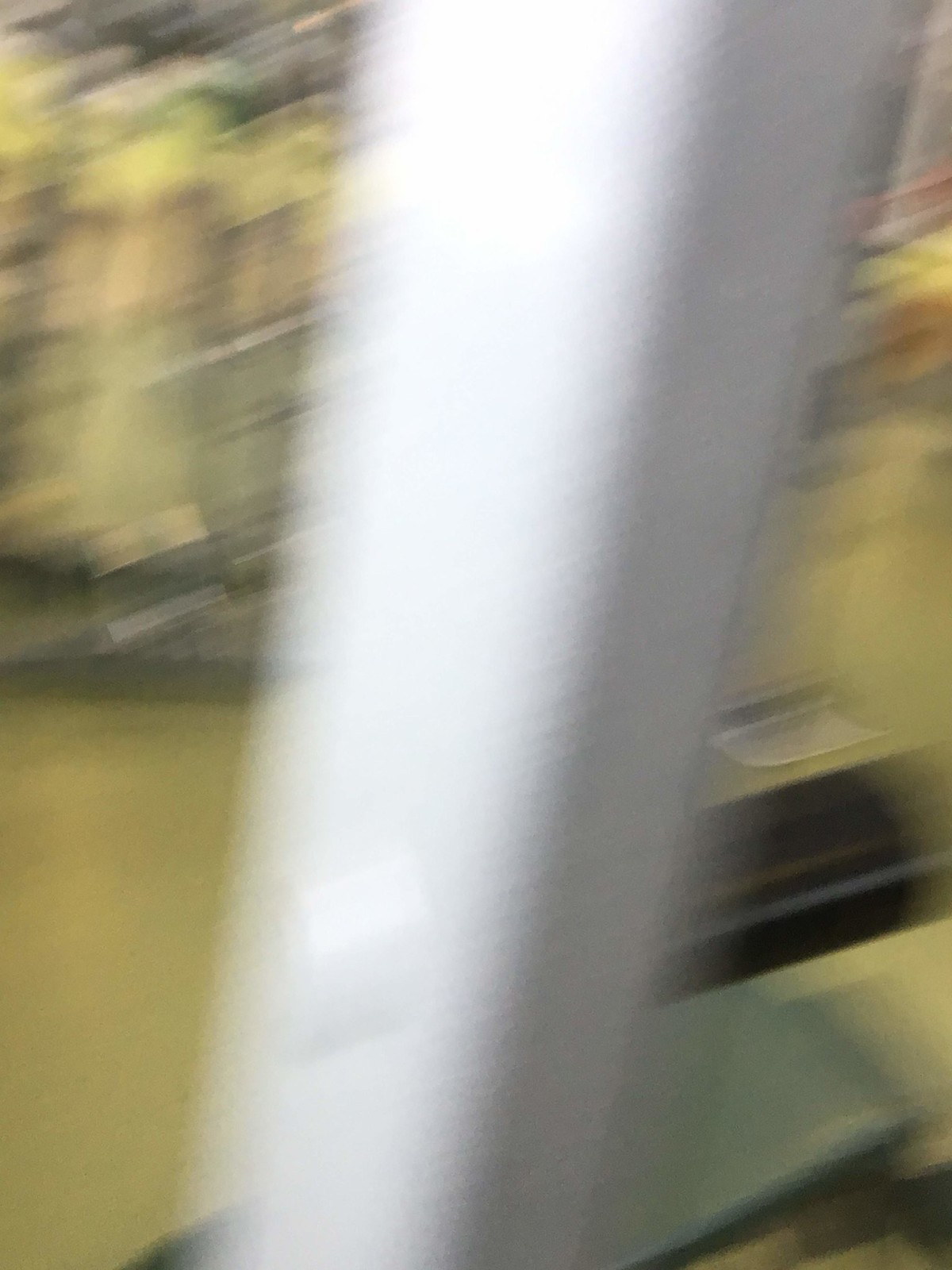The blurry image appears to showcase an outdoor scene dominated by a large, possibly crooked white fixture or stand, which extends from the top to the bottom of the image. To the left, a sequence of colored blurs—starting with yellow, followed by light brown, light green, dark green, and light green again—creates a layered effect. On the right side, there is a prominent white bar, possibly a structural element, that casts a shadow to its right and transitions to a light gray tone. Behind this fixture, various colors blend together, including dark green with a black blur on top, light green, orange, yellow, and pink. The background seems to suggest an outdoor environment with water and greenery, resembling trees or foliage. Additionally, there is mention of potential exercise equipment on the left, but the extreme blurriness makes it difficult to identify the objects precisely.